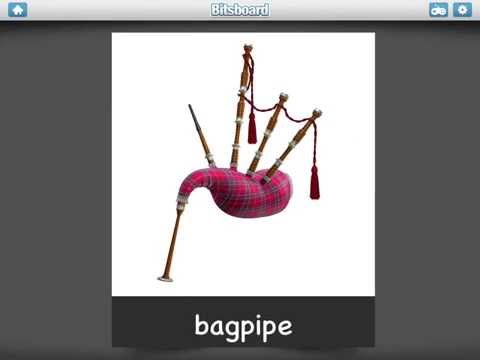The image is likely a screenshot of a computer browser displaying an application or website called Bitsboard. The interface shows a dark gray background with a light gray banner at the top. On the top left, there's a home button, and in the center, the title "Bitsboard" is displayed in white text. On the right side of this banner, there are icons, one resembling a joystick or controller and another that looks like a settings gear.

In the center of the image, there's a large white square containing a picture of red plaid bagpipes, which could also be described as a reddish-purple color. Directly beneath this white square is a narrow black banner extending the same width as the square, with the word "bagpipe" written in white font. The icons at the top are blue, contrasting with the overall grayscale theme of the background.